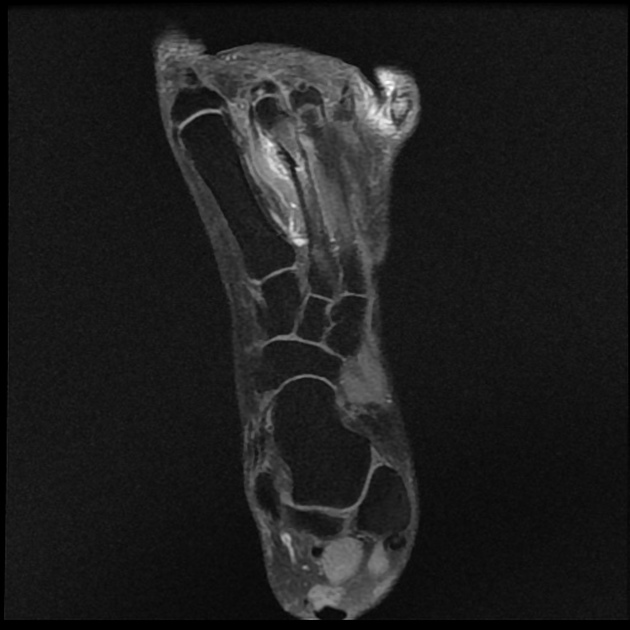The image features a detailed x-ray, dominantly black in the background, presenting what appears to be the right foot due to its soul-like shape and tapered form. The x-ray displays a grainy texture, with the structural focus depicted in varying shades of gray. The overall shape shows a more narrow base, widening at the top, with intricate divisions that resemble bone or cell-like structures. The bones stand out in a prominent dark black against the lighter grayish hues of the surrounding tissue. This central grayish figure, almost resembling a translucent blob, floats within a completely dark square, enhancing the contrast and making the detailed anatomy of the foot's internal structure more prominent. There are no words or additional markings in the image.